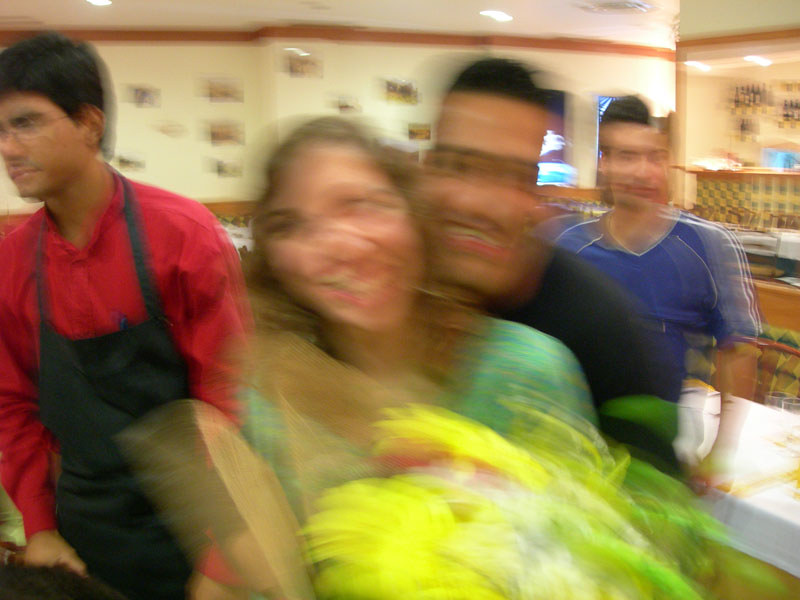The photograph, although blurry, depicts a vibrant moment inside a well-lit restaurant with white walls accented by an orange-brown trim and adorned with various small, framed pictures. In the foreground, a woman and a man are prominently featured. The woman, who has long brown hair and is wearing a blue top over a white shirt, is beaming a large smile while holding a big bouquet of yellow and green flowers. The man behind her, with short dark hair and a black shirt featuring a green stripe on the sleeve, is embracing her affectionately, his face close to hers over her right shoulder. To the left, slightly in the background, stands a man with short brown hair and small-framed glasses, donning a red long-sleeved button-up shirt with a black apron. Notably, a pen is tucked into his right front pocket, suggesting he might be a restaurant staff member. On the right, another man in a blue V-neck shirt with white stripes on the sleeves stands behind the embracing couple, appearing to lean against a table draped with a white tablecloth. The background reveals a bar area adorned with green and white tiles on the front, a wooden top, and wine bottles hanging from the walls. There are also hints of glasses on tables, adding to the casual dining atmosphere of this snapshot. The overall scene captures a lively, intimate moment among friends or family in a cozy, casual dining setting.